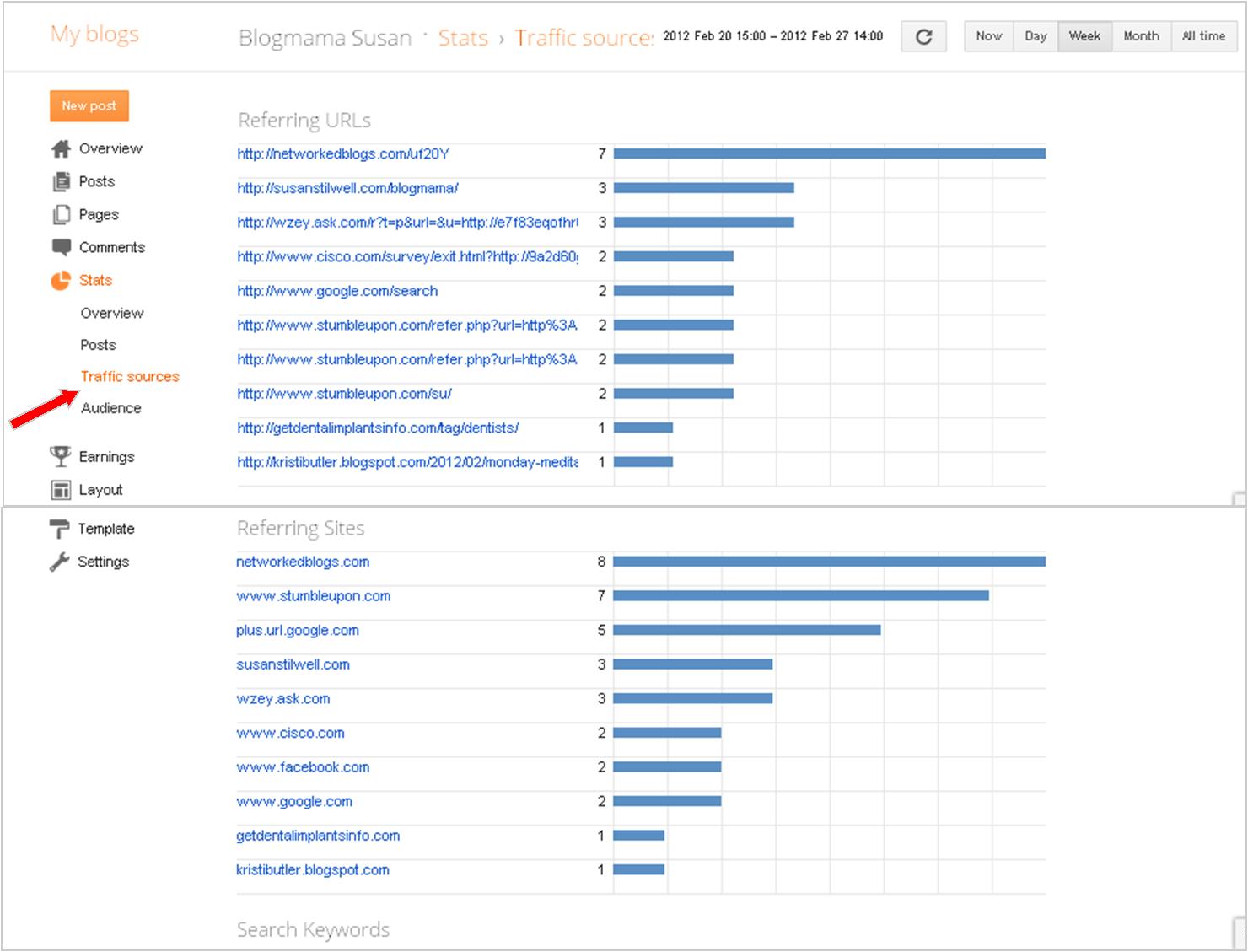Detailed caption: 

The image is a screenshot of a spreadsheet-like page, displaying statistics for a blog titled "Mama Susan." At the top, the page header reads "My Blogs," under which "Blog Mama Susan" is listed. Detailed stats are displayed, including sections for Traffic Source, and a specific date range from February 20, 2012, showing 1500 visits, to February 27, 2012, showing 1400 visits. 

A refresh button is visible, along with time-frame options for data display: "Now," "Day," "Week," "Month," and "All Time." The "Week" option is currently selected, presenting data in a bar graph format.

At the bottom, the graph illustrates referring URLs, with the most referred URL showing a value of 7, represented by a prominent blue line. Subsequent URLs are listed as 3, 3, 2, 2, 2, 2, 2, 1, and 1 respectively. 

Additionally, a section displaying referring sites is present, with the highest value being 8, followed by 7, 5, 3, 3, 2, 2, 2, 1, and 1. The visual differences among the referring sites are conveyed through varying lengths of blue lines, indicating their referral strength.